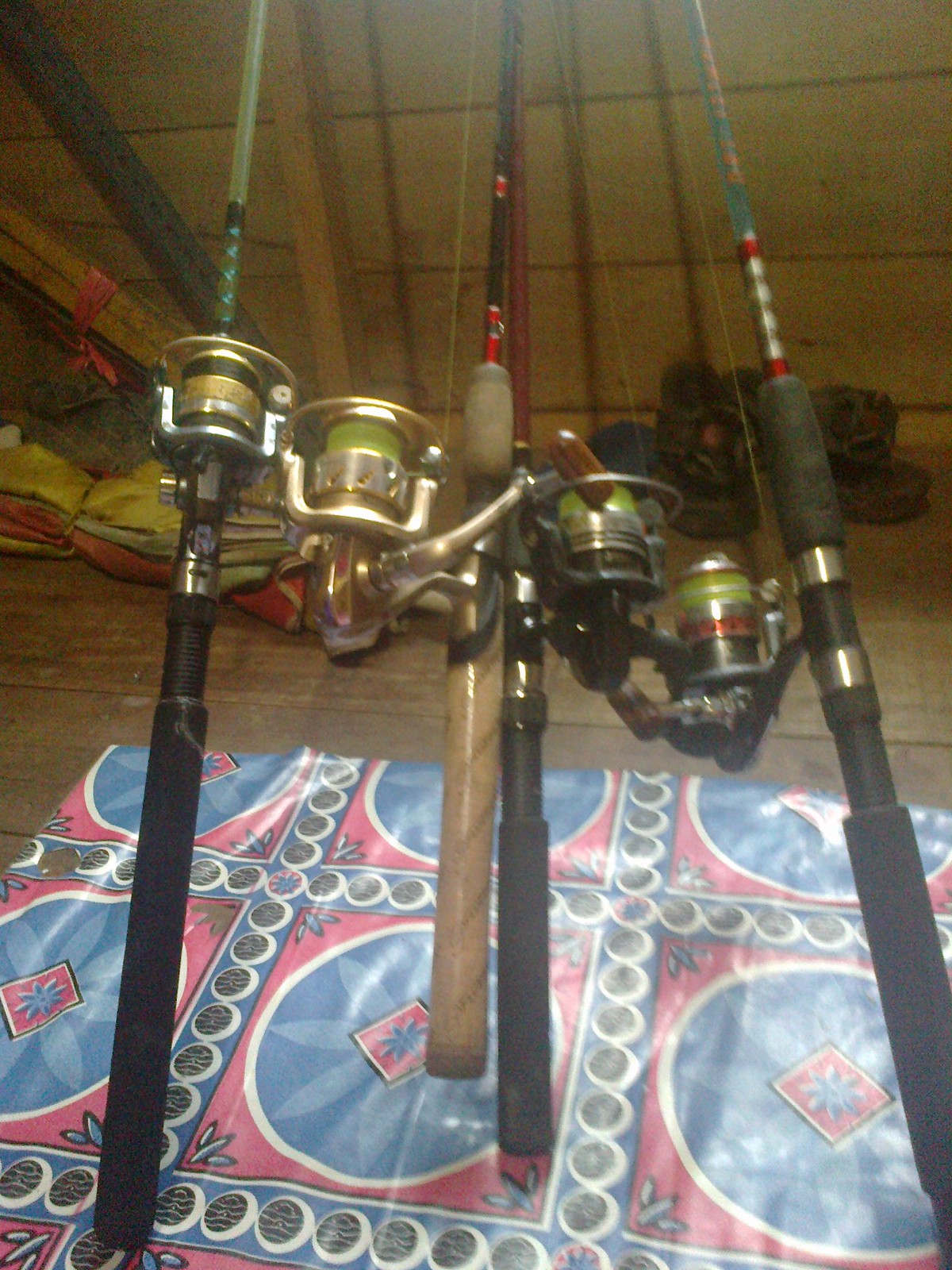This photograph captures four fishing rods prominently featuring their reels, bases, handles, and partial rod lengths, with the tops cut off by the frame. The photo focuses on the variety of reel styles and handle colors: three rods have black handles, while one has a light brown handle. The reels differ in design, with some sporting wooden handles and others metal. The rods are arranged on a folded square fabric adorned with blue, red, white, and black decorative patterns resembling leaves, which sits on a brown wooden surface. The setting appears to be within a wooden structure, perhaps a storage shed or boat, evidenced by the wooden floor and additional visible items like a pair of shoes. All the rods have fishing lines attached and are positioned with their bases on the fabric, leaning against a wall.